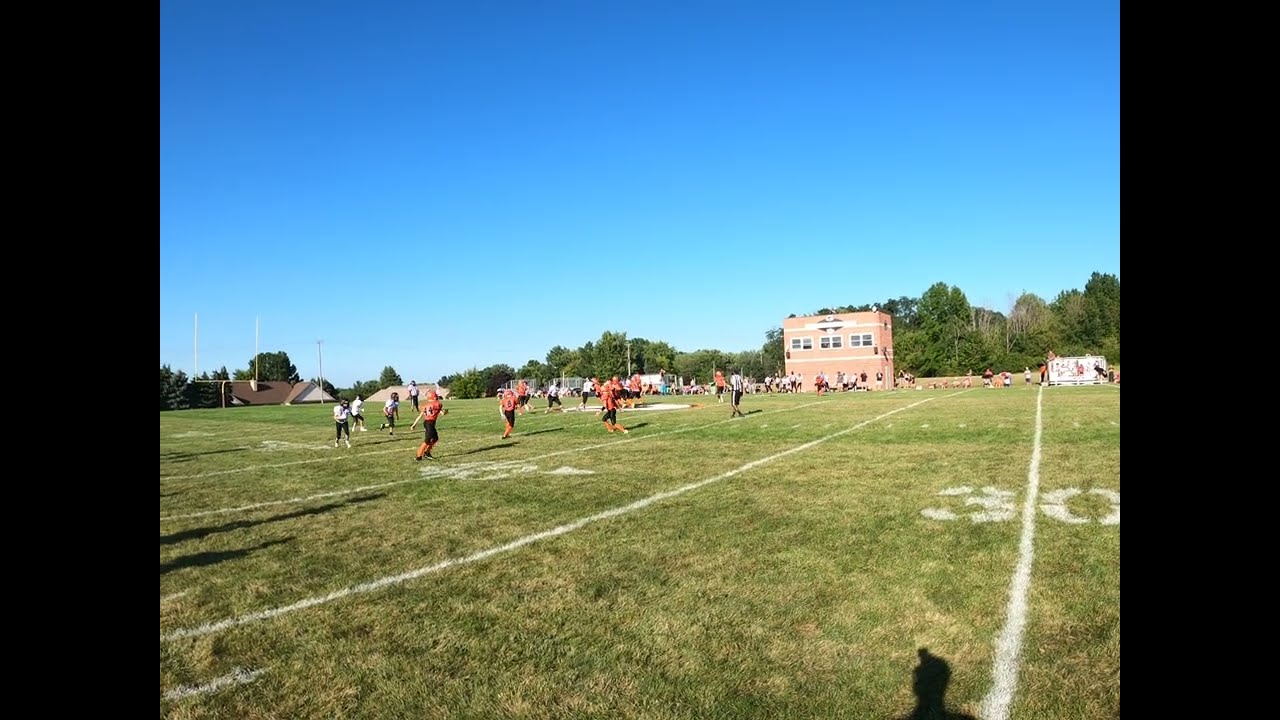The image captures an outdoor peewee football game on a bright, sunny day with a clear blue sky. The green grass field is marked with white yard lines and numbers, and the scene is angled diagonally from the bottom left corner towards the middle of the right edge. The orange team, wearing orange jerseys with black pants, is playing against the white team, adorned in white jerseys with black pants, or potentially blue pants as well. The 30-yard line is visible towards the right side of the image, extending towards the end zone and goal posts on the left. Referees in black and white stripes can be seen officiating the game. Surrounding the field, there are numerous spectators lining the far side. The background includes lush green trees, suggesting a natural setting, and a small, two-story red or brick building with orange hues and white-bordered windows. Additionally, there is a white structure, possibly a scoreboard or announcement board, and hints of a residential area with a house visible further back. A yellow field goal post stands prominently against the vibrant blue sky, completing the picturesque scene.